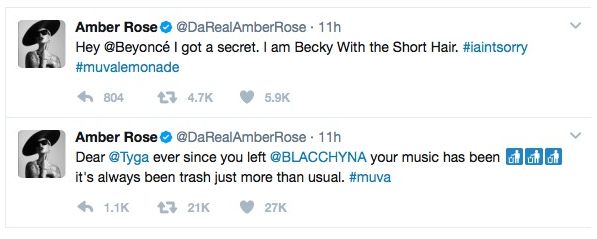The image depicts two social media posts displayed one above the other, both originating from a profile named "Amber Rose." The profile image, which accompanies both posts, is a black and white photograph of a woman wearing a large brimmed hat. To the right of this image, the profile name is written in black text as "Amber Rose," followed by the handle "@TheRealAmberRose." Both posts were made 11 hours ago.

The first post reads: "Hey, @Beyonce, I got a secret. I am Becky with the short hair." This post has garnered substantial engagement, amassing 5.9 thousand likes.

The second post begins: "Dear @Tyga, ever since you left @BlacChyna, your music has been..." The exact sentiment of this post isn't fully captured in this snippet and appears to be cut off in the image.